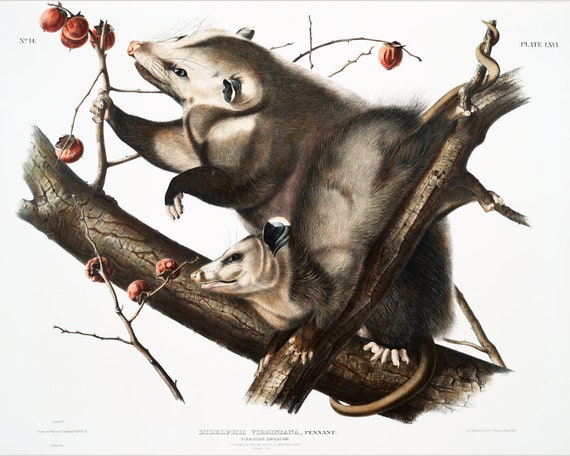The square image features a detailed artistic depiction of two possums positioned on a diagonally placed tree branch against a white background with thin light brown borders at the top and bottom. The larger possum, with dark fur and a white face, appears chubby and has tiny ears, a pink nose with whiskers, and small black eyes giving it a curious yet somewhat mischievous appearance. It is gripping a smaller branch sprouting from the main log with its white claws and mouth, and its tail is wrapped around the branch. The branch contains round, red fruits resembling acorns. Below the larger possum, a smaller possum, similar in appearance but tilted upside down, mirrors the action of reaching for the fruits on a branch, contributing to a dynamic and lively scene.